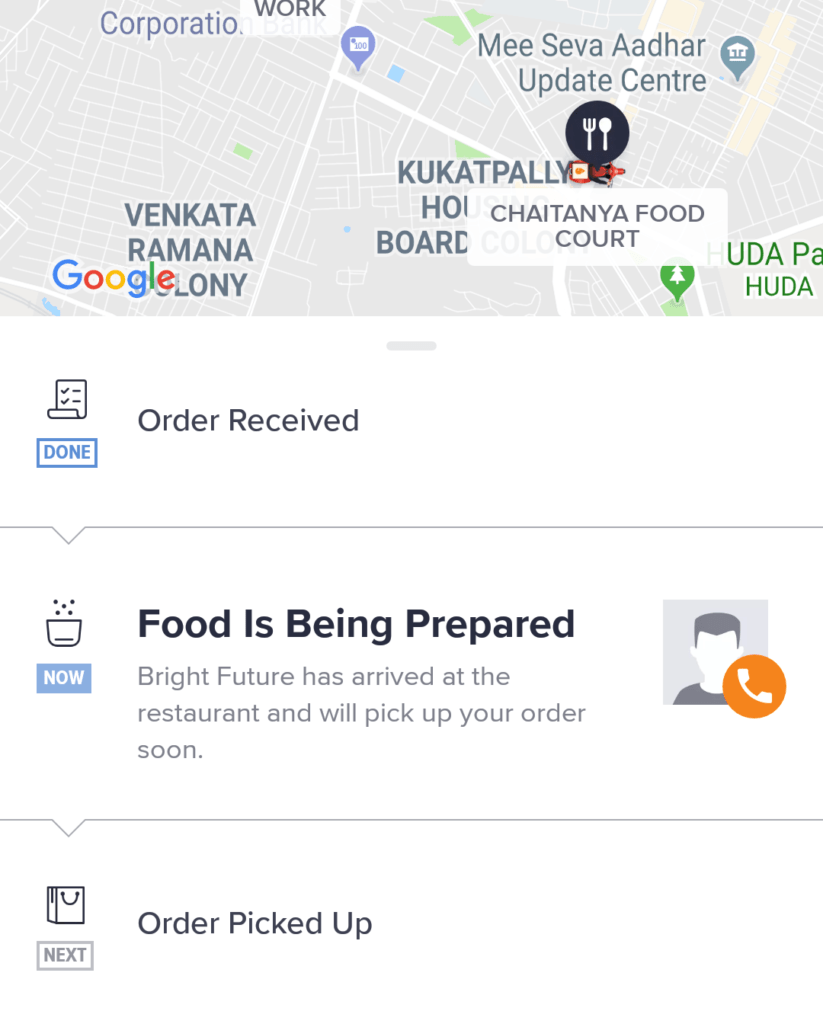The image displays a mobile food order interface. At the top of the screen, a Google Map is visible, highlighting the Chaitana Food Court and the user's workplace, along with various surrounding locations. Below the map, the status "Order Received" is prominently displayed next to a "Done" button.

Further down, a notification indicates that the food is currently being prepared. The text reads, "Bright Future has arrived at the restaurant and will pick up your order soon." Adjacent to this message, there's an outline of a person and an orange button featuring a cellular phone icon, suggesting that it can be used to contact the delivery person.

A logo labeled "Now" signifies the real-time status update for the food preparation. The next step in the process, "Order Picked Up," is represented by a small bag icon, which will be updated once the pickup occurs.

The background of the interface is predominantly white with a detailed map at the top, showcasing different streets and overall area. Various logos, including a fork and a spoon, are scattered across the map, indicating various dining and food-related locations.